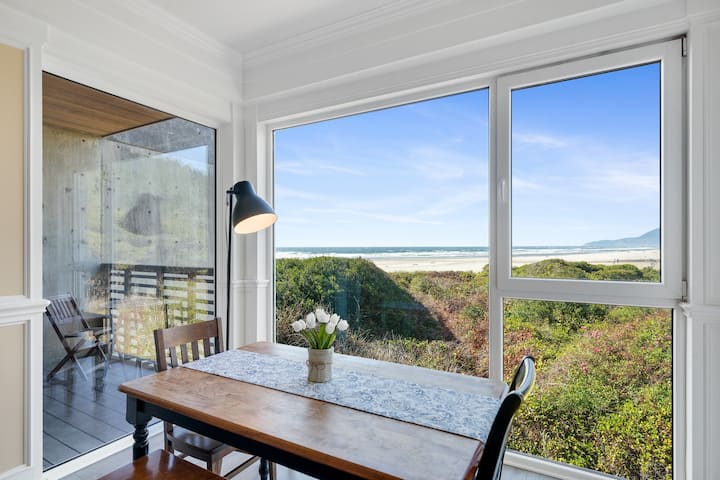The image captures a serene dining nook situated by a large, multi-pane window with a scenic view of a beach. The dining room table, set for two with a table runner and a small pot of flowers, is illuminated by a black standing lamp. Directly behind the table, you see three glass panes offering a breathtaking look at the outside landscape. The largest pane on the left allows a clear vista of the lush, green sand dunes dotted with shrubs and small trees. Beyond the dunes, a white sandy beach stretches out to meet the crashing waves of a seemingly endless ocean. The sky overhead is mostly clear, adorned with a few wispy, fluffy clouds. Adjacent to this seating area, there is a sliding glass door leading to a balcony, which is furnished with a chair and encircled by a railing that separates the interior from the outdoors. This picturesque setting invites you to enjoy a peaceful breakfast while soaking in the stunning coastal scenery.